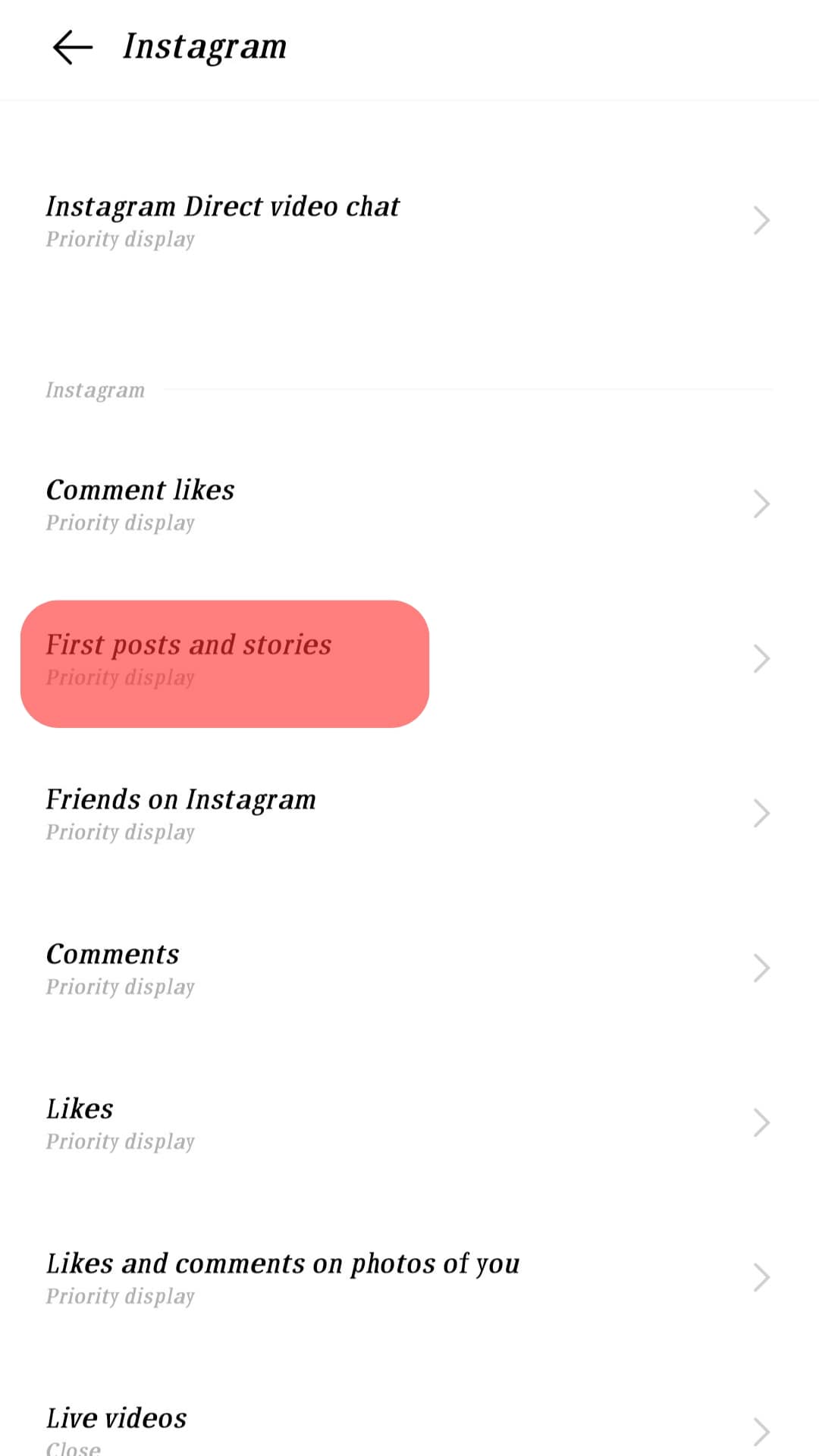A screenshot from a mobile device displays a submenu within the Instagram app. The interface has a clean white background with black text. At the top, the word "Instagram" is displayed, accompanied by a back arrow icon, indicating the option to navigate to the previous page. Below this header are various settings options, each accompanied by right-pointing arrows indicating further submenus.

The list begins with:
1. **Instagram Direct Video Chat Priority Display**
2. **Comment Likes Priority Display**
3. **First Posts and Stories Priority Display** (highlighted in red)
4. **Friends on Instagram Priority Display**
5. **Comments Priority Display**
6. **Likes Priority Display**
7. **Likes and Comments on Photos of You Priority Display**
8. **Live Videos Close**

Each setting in the list suggests a customizable feature, likely related to notification preferences or content prioritization within the Instagram app. The screenshot appears to be from a settings page where users can tweak their interaction preferences on the platform.